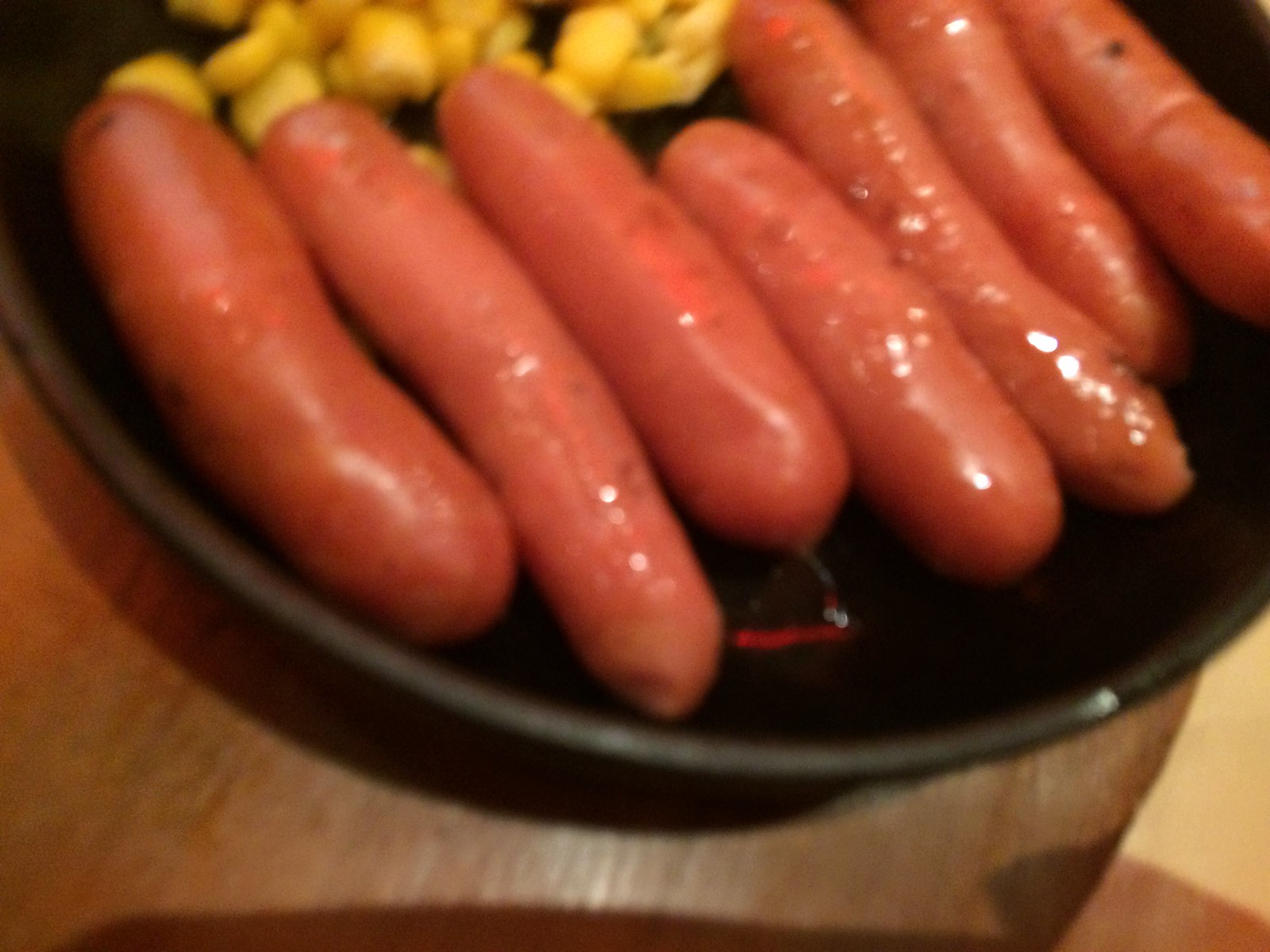In this image, a round cast iron frying pan is seen sitting on a medium wood-grain table or countertop. The pan contains seven sausages of varying sizes, which are slightly fatter than typical hot dogs and have a reddish-brown, shiny appearance, likely from the cooking fat glistening on them. The sausages are arranged closely together and look like they are in the early stages of cooking. Also in the pan, to one side, are yellow kernels of corn, which seem sautéed, adding a splash of color to the dish. The bottom of the pan reveals a mysterious faint red glow or reflection, possibly from a heating element under the wooden surface. The lighting from above creates a reflection on the shiny surfaces of the sausages.